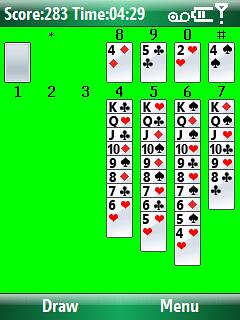A vintage mobile phone screen displays a classic game of Solitaire in progress. The top-left corner shows the current score of 283, with a timer reading 4 minutes and 29 seconds below. The battery indicator reveals two bars remaining, positioned next to the Bluetooth symbol on the top-right. Adjacent to these is an icon with two overlapping circles, resembling a speech bubble.

The Solitaire layout consists of 8 columns, with each column containing a mix of cards. At the very top, the face-up cards include the Four of Diamonds, Five of Clubs, Two of Hearts, and Four of Spades, among others. The tableau features a descending sequence from the Kings of various suits down to the Six of Hearts, Five of Hearts, Four of Hearts, and Eight of Clubs, spread across six rows.

Further down, the screen displays the options "Draw" and "Menu" in the bottom corners. The overall design and layout suggest this game is being played on a small, retro mobile device, reminiscent of early Nokia phones.